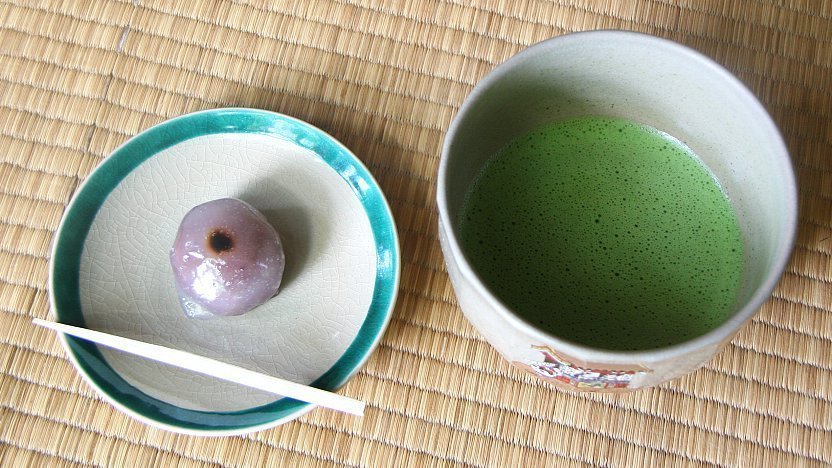The image showcases a meticulously arranged Japanese-inspired meal set on a light brown, woven bamboo mat. To the right, a deep, handleless ceramic teacup holds a freshly poured green tea, evidenced by the small bubbles still floating on the surface. Adjacent to the teacup on the left, a small, white ceramic plate with a teal rim displays a single, exquisite delicacy. This delicacy is a round, purple-hued morsel with a dark red dot at its center, closely resembling a mochi or a traditional bean paste dessert. Resting across the plate is a pair of white chopsticks, likely for handling the featured delicacy. The overall presentation, highlighted by the simple yet elegant ceramic dishes and bamboo mat, suggests a minimalist and traditional Japanese aesthetic.